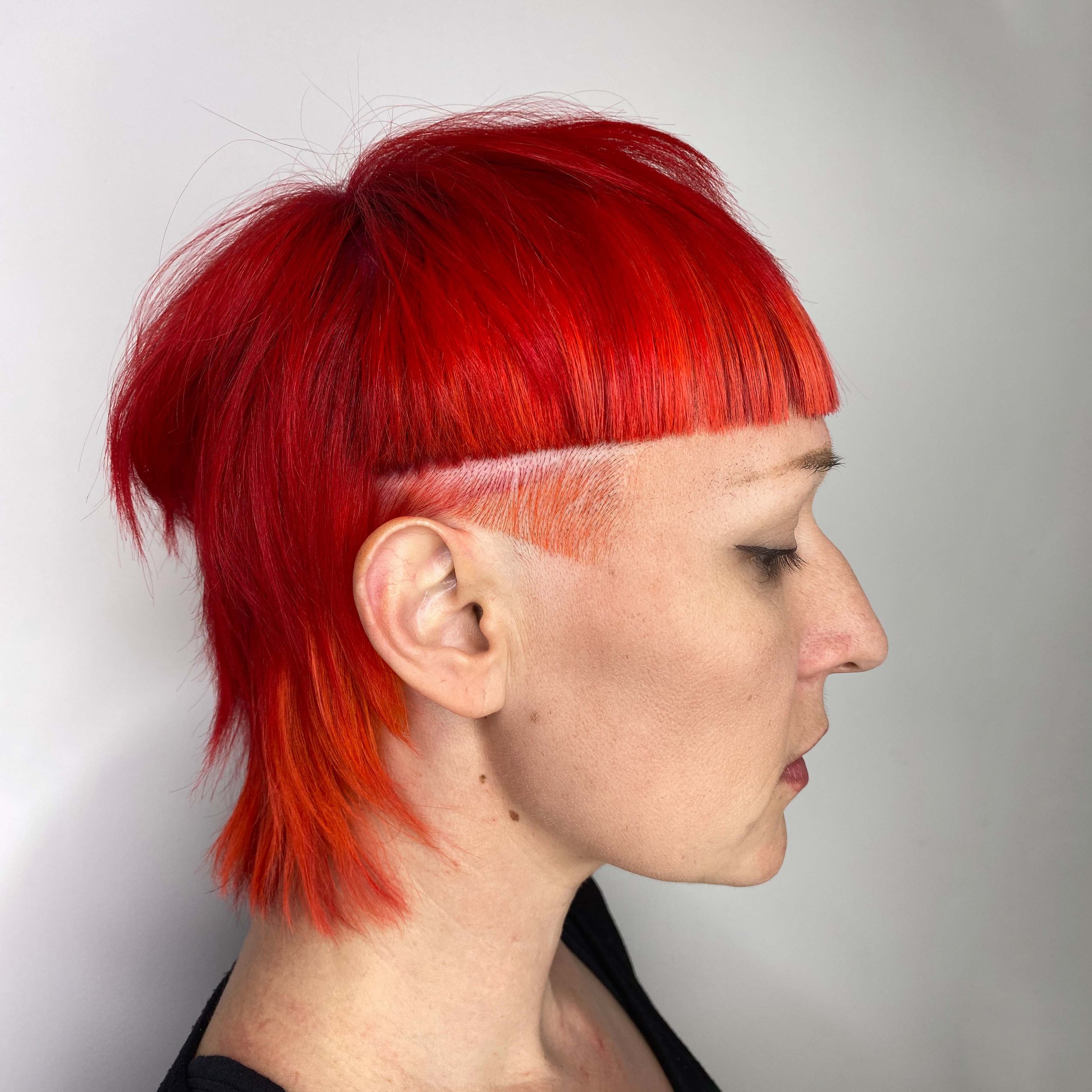This image is a color photograph in a square format, capturing the side profile of a white female model in her late twenties or early thirties. She is standing against an off-white background, looking down towards the right. Her hair is dyed a striking bright orange-red color. The haircut features a mixture of styles: a sharp, straight-across bang at the forehead, transitioning into a layered mullet at the back. The area around her temple and ear is buzzed very tight with artistic precision, blending seamlessly into the longer, slightly messy shag at the top. Her sideburns are almost completely shaved. She is dressed in a black scoop neck top, adding a stylish contrast to her vivid hair. The photo emphasizes photographic representational realism.